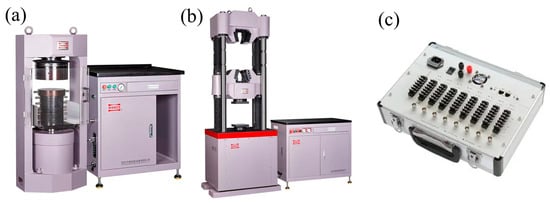The image comprises three detailed shots of industrial machinery set against a white background, each emphasizing complex and sophisticated features likely intended for 3D printing or other industrial tasks. Image A, positioned on the left, showcases a purplish-gray metal machine with a single-door cabinet, topped with a square counter featuring green and red controls and a black counter, all standing on adjustable legs. Adjacent to it is a taller structure with a cylindrical component encased in a matching purplish-gray metal framework. Image B, situated in the center, mirrors the design of the first but with a two-door cabinet below a black counter, also on adjustable legs. This setup includes an extended tower with a central cylindrical object securely clamped within a frame above a square cabinet, accented by a striking red band near the top. Finally, Image C, located on the right, depicts a control device integrated into a perfectly rectangular metal briefcase, characterized by a black handle and two silver buckles. The front panel of this briefcase hosts an array of controls: a row of eight knobs near the handle, nine vertical lines of black controls above, and various smaller, color-coded controls in black and red at the top.